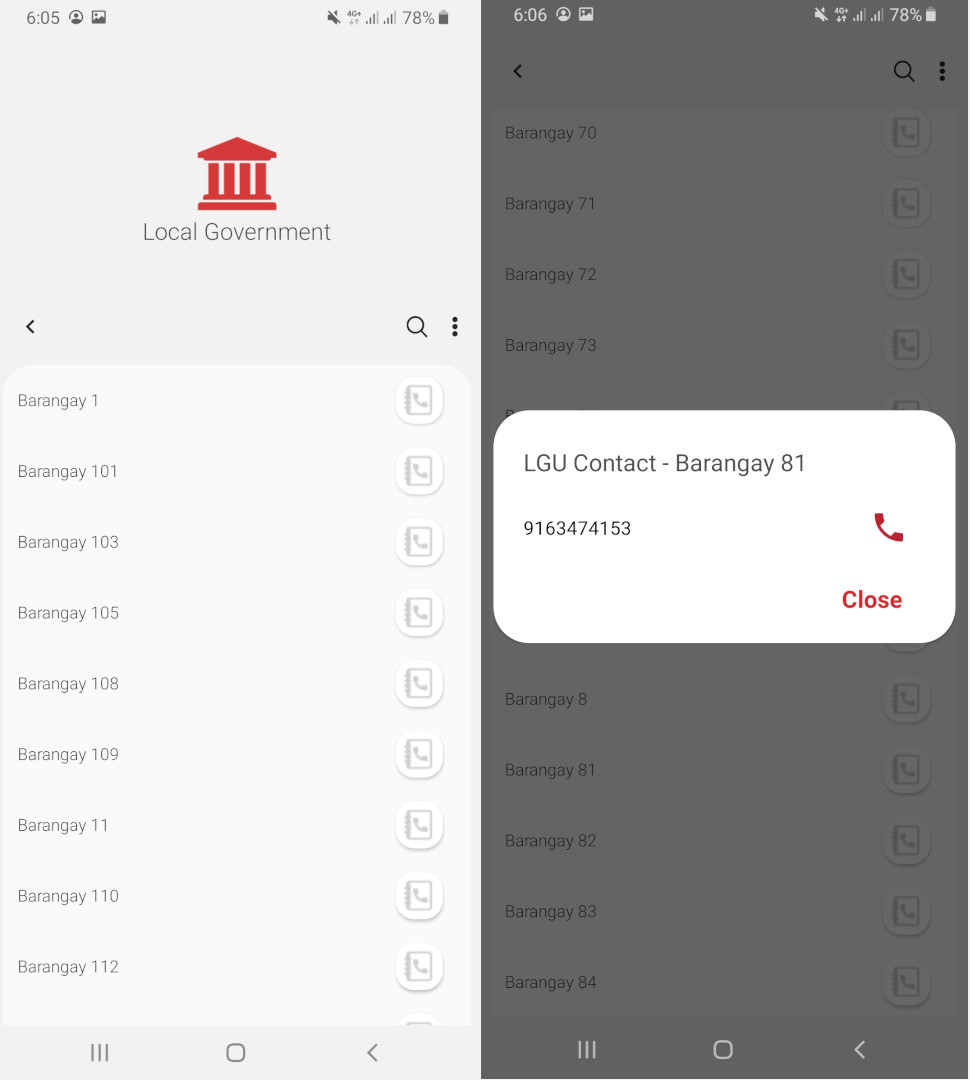Left Screenshot: Shows a smartphone display at 78% battery, featuring a screen with a light gray background. It is titled "Local Government" and includes an icon resembling a classic Federalist-style building. There is a comprehensive list of at least nine barangay names with phone icons next to each name indicating contact availability. The visible barangays are: 1, 101, 103, 105, 108, 109, 11, 110, and 112.

Right Screenshot: Depicts the same smartphone with a dark gray background. It appears that an item from the list on the previous screen has been selected, triggering a pop-up dialog. The pop-up displays the title "LGU Contact Barangay 81" along with the contact number "916-347-4153" accompanied by a red phone icon. Below, there is a "Close" option available to exit the dialog.

Combined Caption: A dual-screen smartphone display at 78% battery shows an interface for contacting local government barangays. The left screenshot features a light gray background with a list of nine barangays, each with a phone icon symbolizing contact capability. The right screenshot displays a dark gray background where a user-selected barangay name (Barangay 81) prompts a pop-up dialog containing specific contact information (916-347-4153) and a red phone icon, with an option to close the dialog at the bottom right.